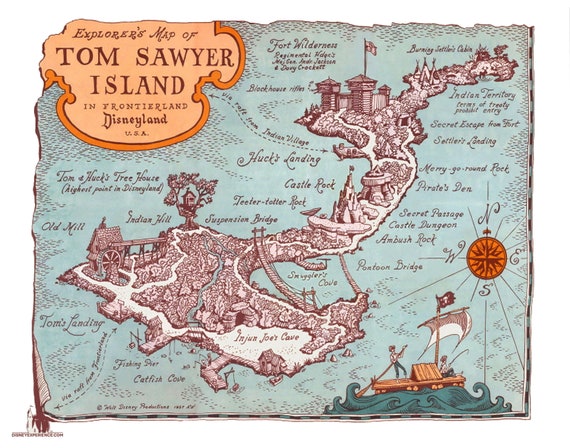This detailed and colorful map of Tom Sawyer Island at Disneyland appears to be commercially produced, possibly through computer generation or hand-drawing. At the top of the map, the text prominently reads "Tom Sawyer Island, Disneyland," indicating its specific location. The map showcases the island set against a vibrant blue background, enhancing the contrast with the island's reddish and white tones.

Central to the map is an intricate depiction of Tom Sawyer Island, a long-standing attraction at Disneyland. Various points of interest on the island are illustrated, providing a comprehensive guide for visitors. To the far right, an orange compass is depicted, clearly marking the directions north, south, west, and east, adding navigational context to the map.

At the bottom of the image, there is a detailed drawing of a long sailing ship, possibly a pirate ship, complete with a flag at the top and a prominent white sail. This ship adds a nautical theme to the map, enhancing its visual appeal and aligning with the adventurous spirit of Tom Sawyer Island.

Overall, the map is a visually engaging, well-integrated representation of the Tom Sawyer Island attraction, offering a detailed guide to its various features and enhancing the visitor experience.